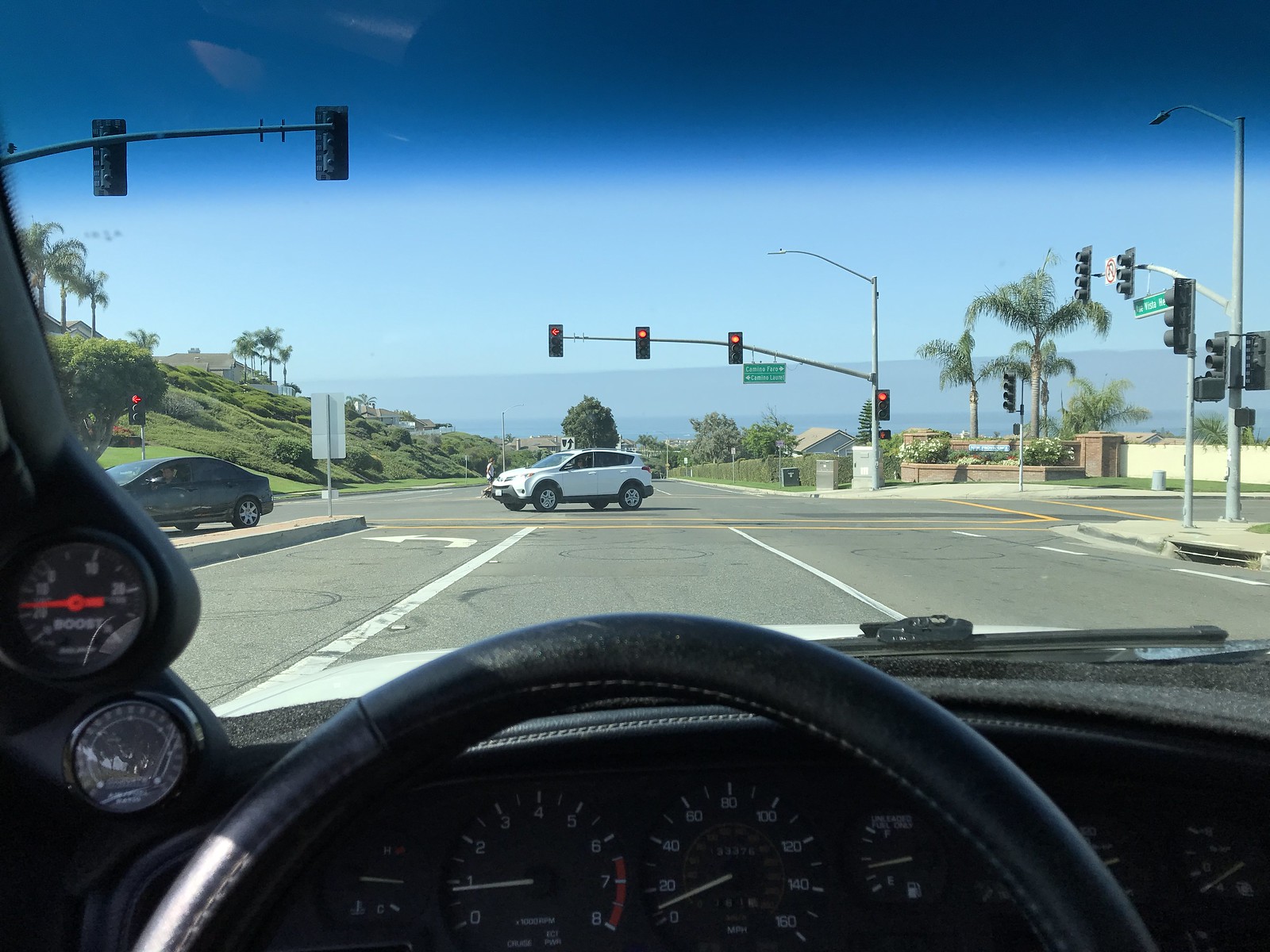This image, taken from the driver's seat of a car, showcases a scene through the windshield. In the foreground, a white SUV is captured mid-turn, making a left maneuver in front of the stationary vehicle. Ahead, a traffic light displays a vivid red signal, indicating a stop. In the distance, a flat-topped mountain rises against a clear, azure sky, free of clouds. Below the mountain, a serene body of water stretches out, reflecting the clear day. On the right side of the frame, a cluster of tall palm trees with green fronds sways gently. Additional traffic signals are visible on the right, adding context to the urban setting. The overall ambiance is one of calm and clarity, emphasized by the bright, unobstructed daylight.